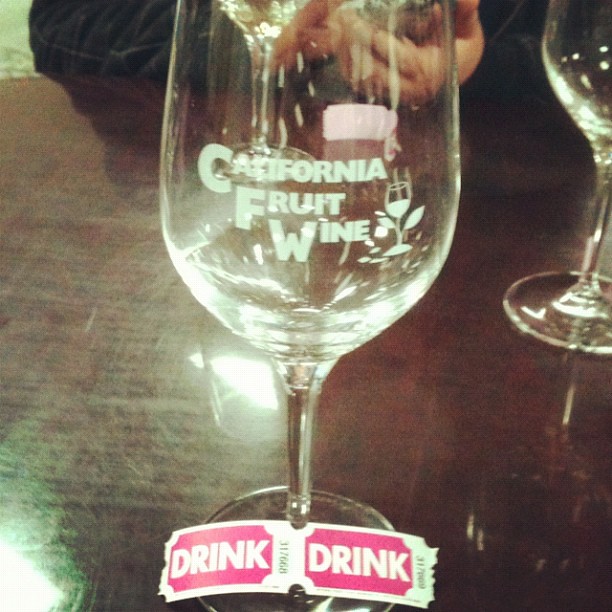The photograph captures a striking scene of a shiny, dark brown table, possibly lacquered wood, reflecting the camera's light at its center. The focal point is a stemmed glass with the words "California Fruit Wine" etched prominently on the bowl, accompanied by a logo depicting a wine glass adorned with a couple of leaves. The large letters "CFW" stand out on the glass. Resting at the base of the glass are two pink carnival-style tickets with white text that reads "drink". These tickets are intact and laid across the bottom of the stemware. Two more empty glasses are visible; one to the upper middle left and another faintly seen through the main glass against the backdrop. At the very top of the image, a person dressed in a long-sleeve black garment can be seen, with their hands resting on the table, contributing a subtle human element to the still life composition.